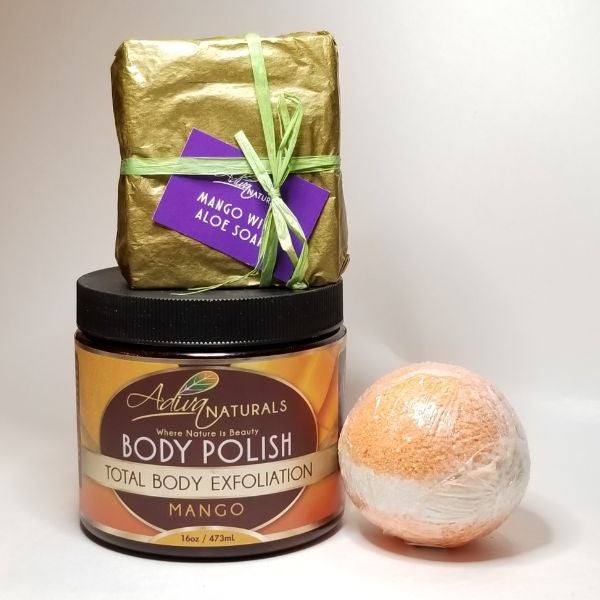This indoor, full-color photograph features three distinct cosmetic items meticulously arranged on a white countertop against a light gray wall. The first item, situated in the upper left, is a bar of soap wrapped in shimmering gold foil, adorned with a green ribbon, and attached to a purple card reading "Mango Aloe Soap." Below this soap is a cylindrical plastic jar of Advera Naturals Body Polish, characterized by its black lid and an orange label with light yellow and white text stating "Total Body Exfoliation Mango." Lastly, on the right side of the composition, there is an orange exfoliating ball with a rough texture, encased in plastic, featuring a white stripe around its middle. The illuminating artificial light highlights the thoughtful staging of this vertically rectangular image, enhancing the details and colors of the products displayed.